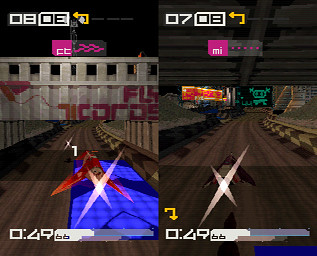A screenshot from a video game features a split-screen display, showcasing two distinct yet parallel scenes. Both screens, located on the left and right sides, depict high-speed fighter jets racing along a track. Each jet is propelled by a bright white star-like flash emanating from its rear, emphasizing their speed. The left screen shows a fighter jet approaching a concrete wall adorned with red writing, suggesting an impending turn or obstacle. In contrast, the right screen offers a clearer path ahead, revealing digital boards displaying black backgrounds with green, creature-like characters. Both screens prominently display the number '49' at the bottom, possibly indicating the player's progress or position in the race.